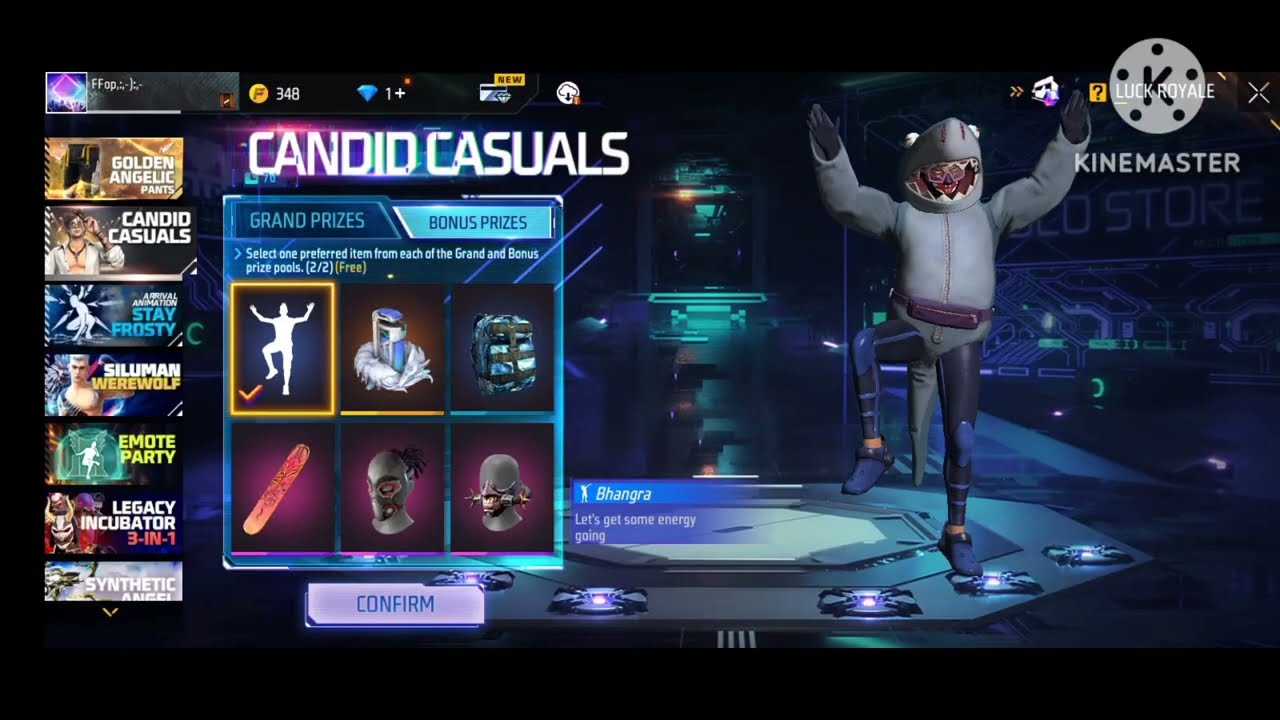The image is a screenshot from a video game. In the top-left corner, there's an elaborate menu displaying several options: Golden Angelic Pants, Candid Casuals (which is checked off), Stay Frosty, Suleiman Werewolf, Emote Party, Legacy Incubator 3-in-1, and Synthetic Arms. The section for Candid Casuals shows six potential prizes, consisting of different helmets, a snowboard, and two face masks, with an option to pick two and confirm the selection. 

On the right-hand side of the screen, a character dressed in a shark suit is standing on one leg, poised on a platform that appears to be a stage or a dance pad. The shark suit includes a gray shirt, visible through the costume, dark-colored pants with knee pads, and blue pants. The backdrop features metallic, shiny circles suggestive of an octagonal dance floor. Above the character, in the top-right corner, the word "KINDMASTER" is visible in white font alongside a grey disc that has five holes and a black "K" in the middle.